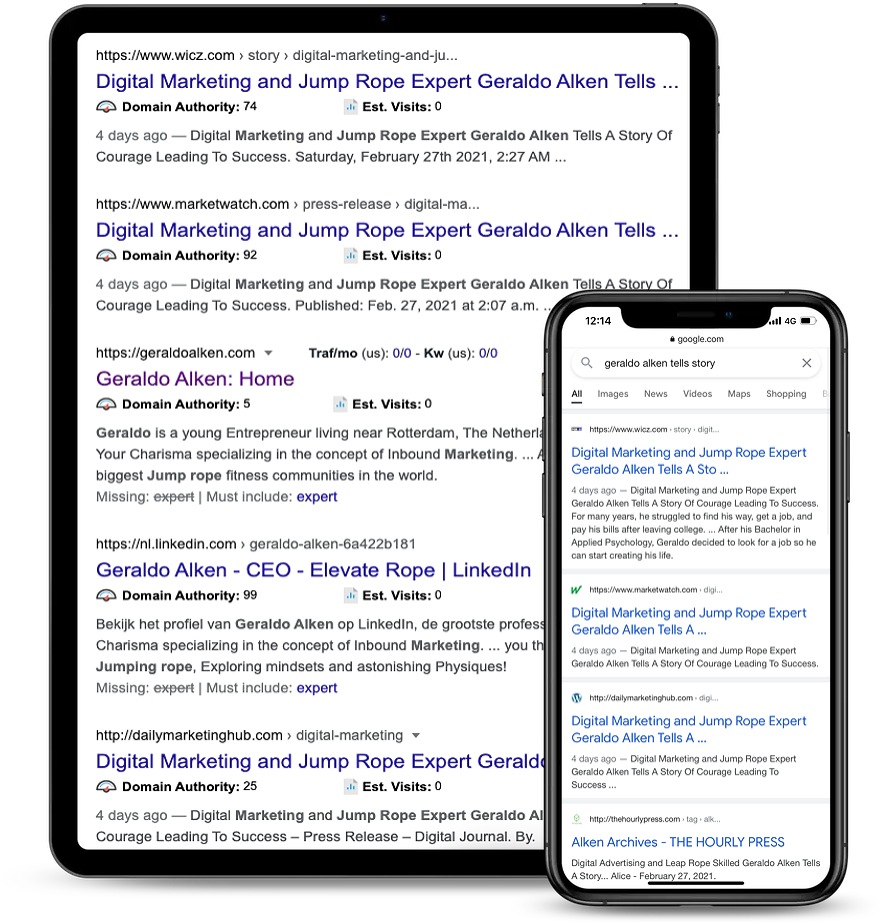A close-up image shows a black tablet and a black smartphone partially covering its screen. The tablet's screen displays a web page with the URL "www.wixi.com," featuring search results for "Gerardo Alcantel Story." The search results include multiple entries about Gerardo Alcantel, identified as a Digital Marketing expert and Jump Rope Athlete. 

The smartphone screen, which overlaps the tablet, also shows a similar web search. The search bar at the top reads "Google.com," and the query "Gerardo Alcantel Story" is visible. Below this, tabs for different search categories such as "All," "Images," "News," "Videos," "Maps," and "Shopping" appear, with "All" being underlined, indicating the active tab.

The search results include:
1. "Digital Marketing, Jump Rope Expert, Gerardo Alcantel" from MarketWatch.com, four days ago.
2. Another entry from "DailyMarketingHub.com" displaying similar information.
3. Gerardo Alcantel's website, which appears in the search results as "Gerardo Alcantel - Home."

The image captures the interface's detailed design along with partial and full URLs, emphasizing the multiple mentions of Gerardo Alcantel's professional roles in digital marketing and jump rope expertise.